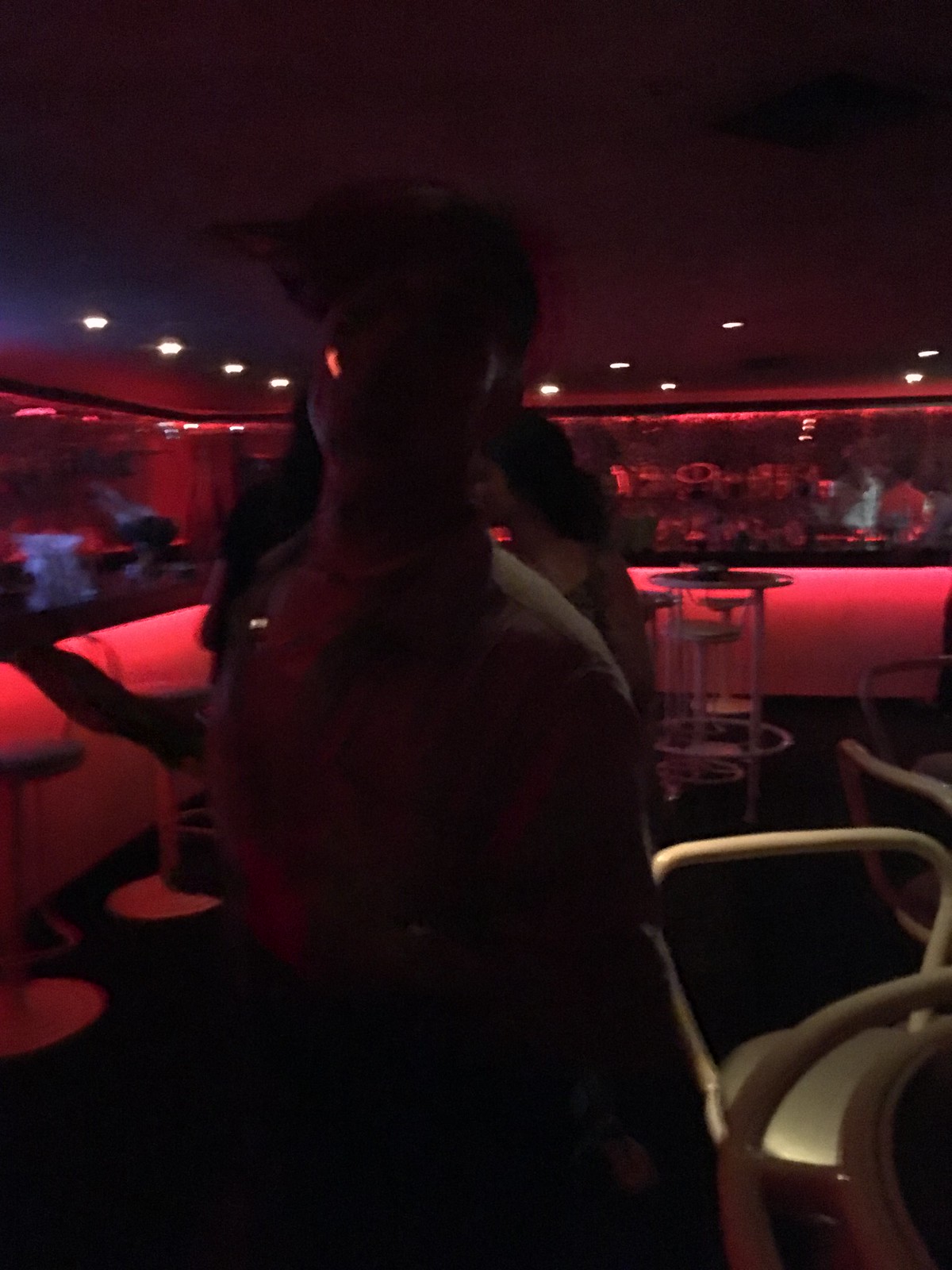This photograph, taken in vertical portrait mode, captures a dimly lit, club-like restaurant or lounge with a distinctly moody ambiance. Central to the image is a man walking towards the camera, his wavy dark hair and indistinct facial features veiled by the low light. The background features an L-shaped bar highlighted by a red underglow, flanked by white stools. Above the bar, an overhead red hue casts a warm, shadowy light, enhancing the atmosphere. To the right, partially cropped by the photo's margins, stands a white circular table and a white chair. The overall lighting is dominated by pinkish tones, with some track and headlight illumination overhead. The carpet in the foreground is dark, adding to the shadowy, intimate feel of the setting. Additionally, a man, possibly the same, is noted to have a broad chest, shoulders, long-sleeved shirt, and a cap from which two bushy ponytails extend. He appears to be gesturing, possibly engaged in conversation, contributing to the lively, yet obscure essence of the photograph.